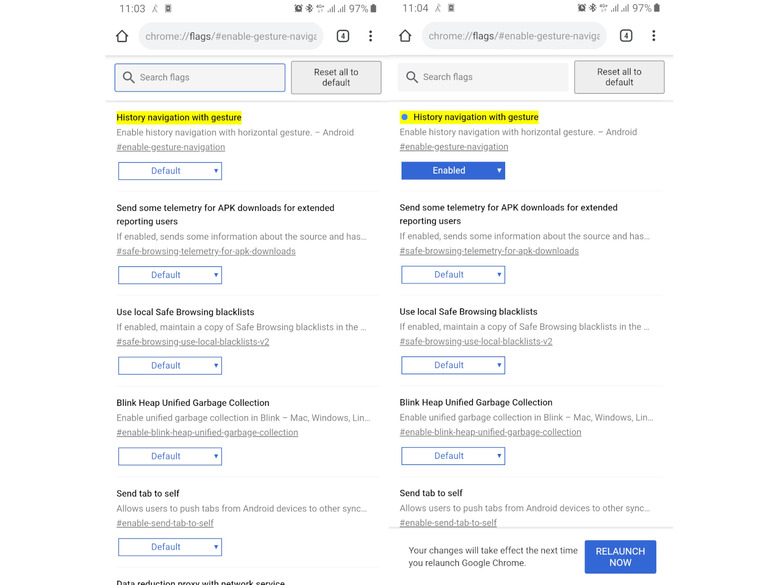This image features two side-by-side mobile screenshots displaying the same web page with different settings adjusted. Both screenshots have a white background with an address bar centered at the top exhibiting the truncated URL "Chrome flags enable gesture navigate...". Below the address bar, there is a rectangular search field containing a magnifying glass icon on the left and a "Reset all to default" button in gray on the right.

Prominently highlighted in yellow below the search field is the option "History navigation with gesture." In the left screenshot, a drop-down box beneath this option is set to "Default." In contrast, the right screenshot displays the same option, still highlighted in yellow, with an additional blue dot on the left side and the drop-down box indicating the setting has been changed to "Enabled." Additionally, a "Relaunch now" button in blue is visible at the bottom right of the second screenshot, indicating that the modified settings can be applied immediately by relaunching the browser.